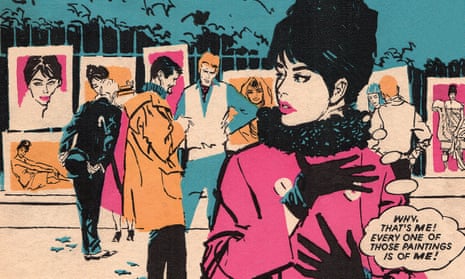This image, reminiscent of a 60s or 70s comic book or old magazine, is a colored cartoon panel rendered in basic shades of pink, blue, yellow, black, and white. It features a rectangular frame, about three inches wide and two inches high, capturing a scene in a gallery setting. The ground in the lower corners is an off-white color, leading up to a blue wall adorned with framed paintings.

At the forefront on the right, from the waist up, stands an elegant young woman with an updo of black hair, pale skin, and pink lips. She is dressed in a pink coat with a black collar and black gloves. A thought bubble emerges from her head, saying, "Why, that's me. Every one of those paintings is of me."

Behind her, four men observe the array of paintings—about eight in total—most featuring backgrounds in purple and orange hues, with some being mere sketches while others are more detailed. These paintings prominently feature the woman herself, aligning with her realization. The setting appears to be a street fence repurposed as a gallery display, filled with life and texture as people engage with the artworks.